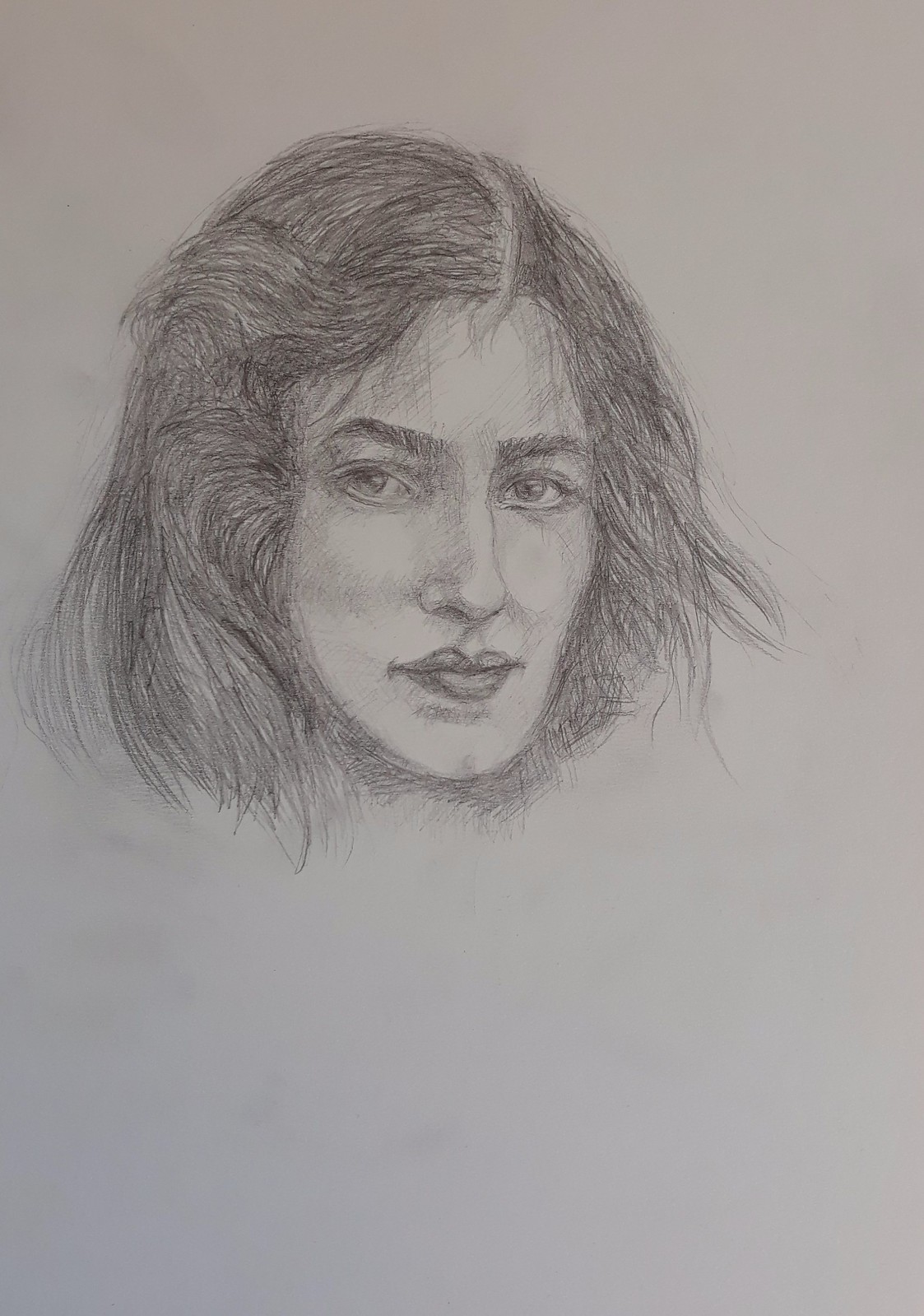A detailed black-and-white sketch depicts a woman's face, artistically rendered on an 8.5 by 11-inch plain piece of paper. Positioned toward the top left of the sheet, the woman's shoulder-length hair, featuring short bangs swept to the side, frames her face. Her thick, distinct eyebrows add character to her expression, while her full, well-defined lips form a subtle half-smile. Detailed shading beneath her lips enhances the minor cleft in her chin, adding depth to the sketch. The woman's nose is long with a gently rounded tip. Her almond-shaped eyes, illustrated to appear light in color, gaze thoughtfully off to the side, contributing to the intriguing composition of the portrait.